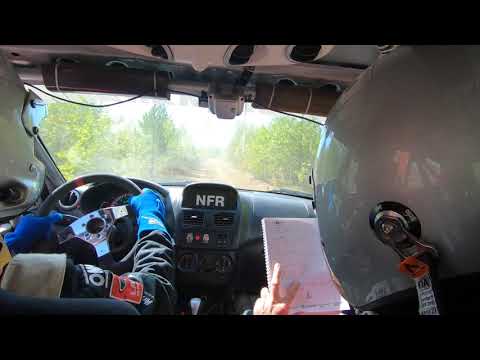Captured from the backseat, this detailed photograph offers an immersive view inside a rally car, likely taken from a video screen given the black borders on the top and bottom. The driver, seated on the left, grips the steering wheel with blue-gloved hands, his full race gear complete with a white helmet. Beside him on the right, the navigator in a gray helmet consults a notebook, his hand near the AC controls of the specially modified dashboard filled with gauges and roll cages. The car is driving on a dirt path through a sunlit forest, as visible through the windshield, with vibrant shades of green from the trees contrasting against the bright sky. Prominently displayed on the center of the dashboard is the 'NFR' logo on an infotainment screen, adding to the high-tech atmosphere of this race day in the woods.